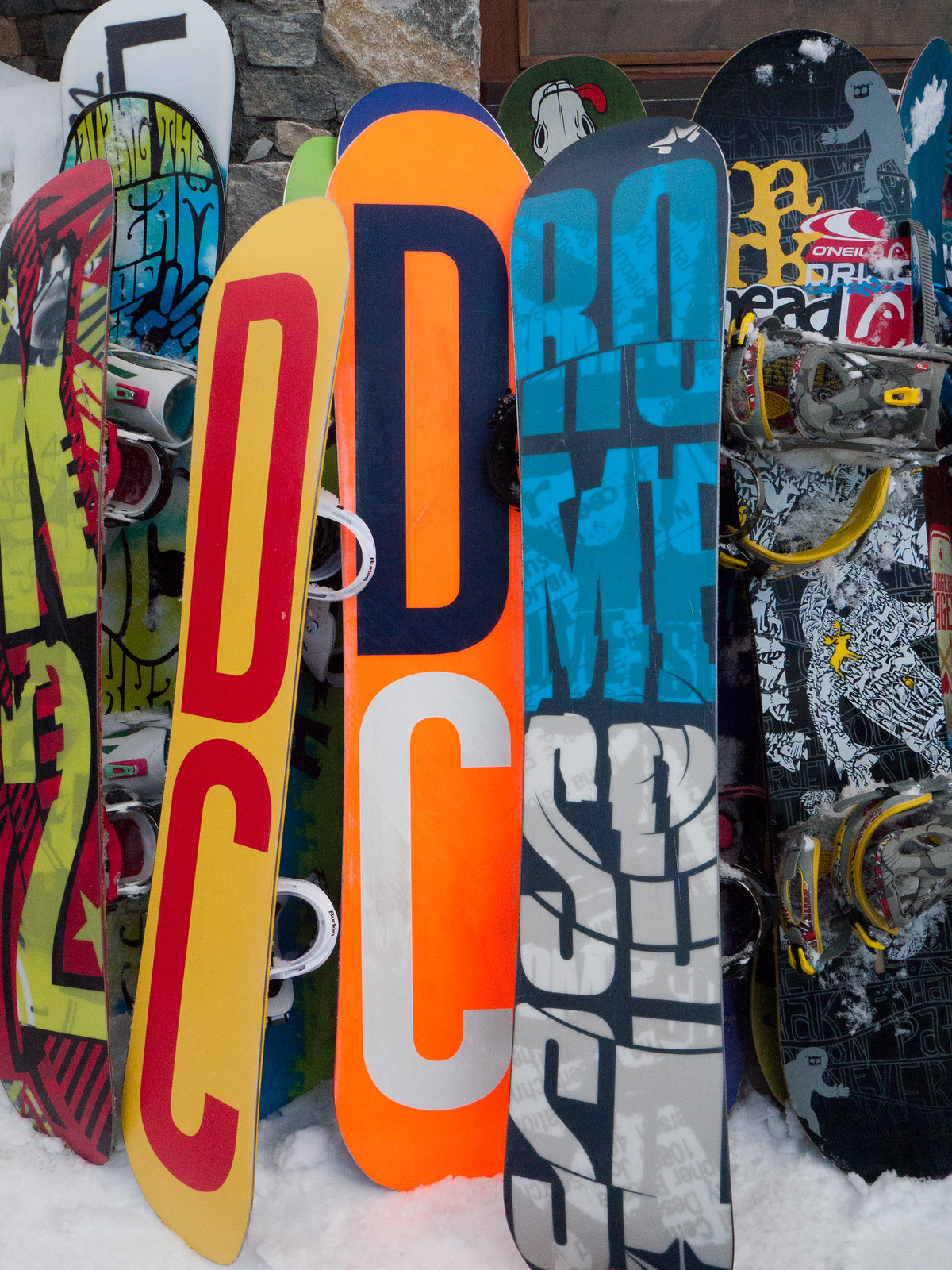This detailed photograph, taken outdoors at what appears to be a ski resort, features 11 snowboards prominently displayed against the backdrop of a stone building, which likely serves as a ski lodge. The ground is blanketed in snow, emphasizing the wintry setting. The snowboards are artfully arranged, leaning upright against the lodge wall, showing off a colorful array of designs. 

On the far left of the image, there is a primarily red snowboard adorned with bold yellow lettering that spells out "K2." Moving to the right, a bright yellow snowboard catches the eye with large red letters, "DC." Adjacent to it is a vibrant orange snowboard featuring a blue "D" and a white "C." A dark blue snowboard follows, showcasing the word "ROME" in blue letters, with "SDS" partially visible beneath in light green and white lettering. On the far right, a predominantly black snowboard stands out with its mix of red lettering at the top and intricate graphic designs at the bottom.

Additionally, part of a window with dark coffee brown wooden framing peeks into view on the upper right side of the building, adding a rustic charm to the scene. The rich variety of colors and patterns on the snowboards, combined with the snowy, picturesque setting of the ski lodge, make this an inviting image for winter sports enthusiasts.